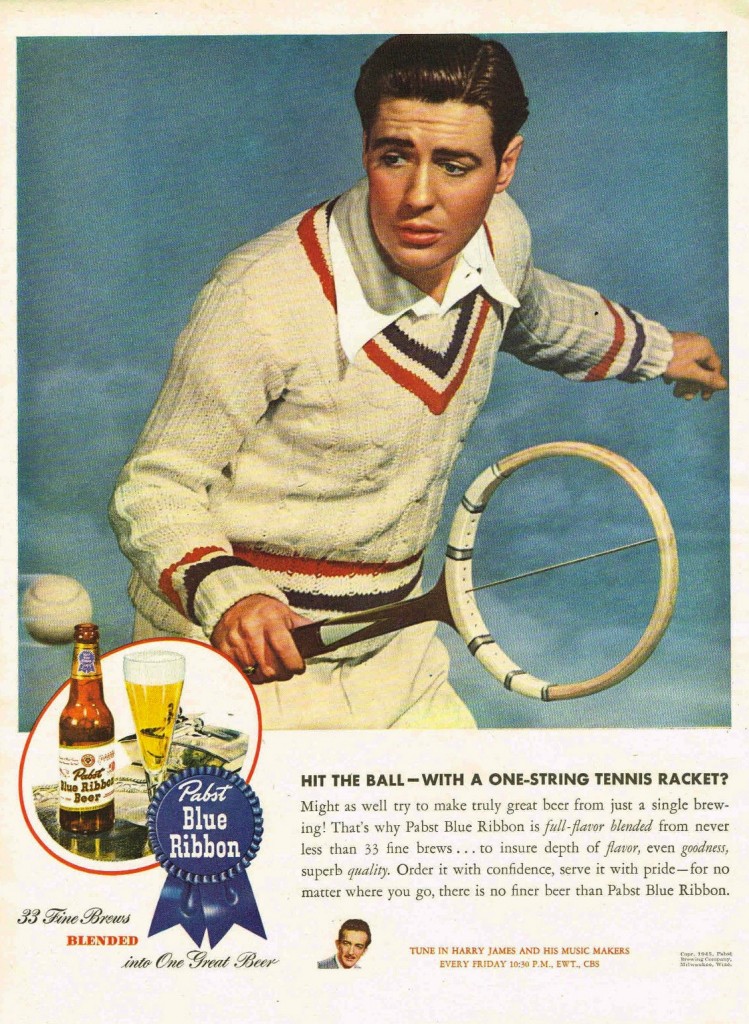The vintage advertisement, likely from a magazine or newspaper, showcases a dynamic image of a man playing tennis. The man, wearing a cream sweater adorned with blue and red stripes on the neck, sleeves, and waistband, pairs it with a white collared shirt and tan pants. He is focused intently on a tennis ball approaching from the left side, poised to hit it with a highly unusual vintage wooden tennis racket featuring just a single string. Beneath this engaging image, the ad captures the essence of its time, cleverly comparing the challenge of playing tennis with a one-string racket to the dedication required to craft a truly exceptional beer from a single brewing process. This theme is reinforced by the prominent display of a Pabst Blue Ribbon beer bottle and a filled glass, accompanied by the brand's iconic blue ribbon logo. Additional text at the bottom encourages readers to "Tune in to Harry James and his Music Makers every Friday," adding a cultural touchpoint to the nostalgic visual.